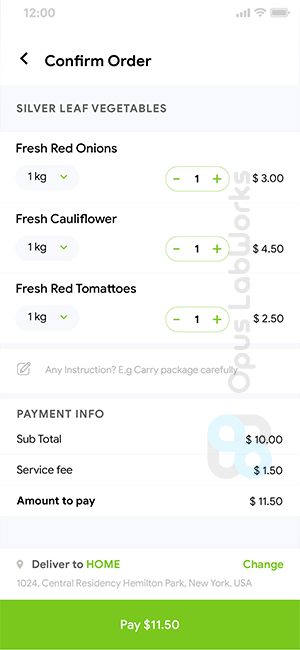**Image Description: Detailed Order Confirmation Screen**

The image displays a screenshot of an order confirmation page against a white background. At the top of the screen, grey text indicates a timestamp marked "12", with status indicators on the right-hand side showing full cell service, full Wi-Fi connectivity, and a fully charged battery.

Below this, there is a black arrow pointing right, accompanied by the text "Confirmed Order". Underneath, grey text reads "Silver Leaf Vegetables", followed by a list of ordered items in black text: 

- Fresh onions, 1 kilogram, $3.00
- Fresh cauliflower, 1 kilogram, $4.50
- Fresh red tomatoes, 1 kilogram, $2.50 

In grey text, an optional instruction field suggests "Any instructions, e.g. carry package carefully". This is followed by black text listing the payment details:

- Subtotal: $10.00
- Service fee: $1.50
- Amount to pay: $11.50

A green text "Deliver to home" option appears, with a "Change" link on the right side. At the bottom of the screen, a prominent green button with white text states "Pay $11.50". The overall context comments on the affordability and convenience of the vegetable delivery service, highlighting the value for fresh produce at 1 kilogram each plus a service fee.